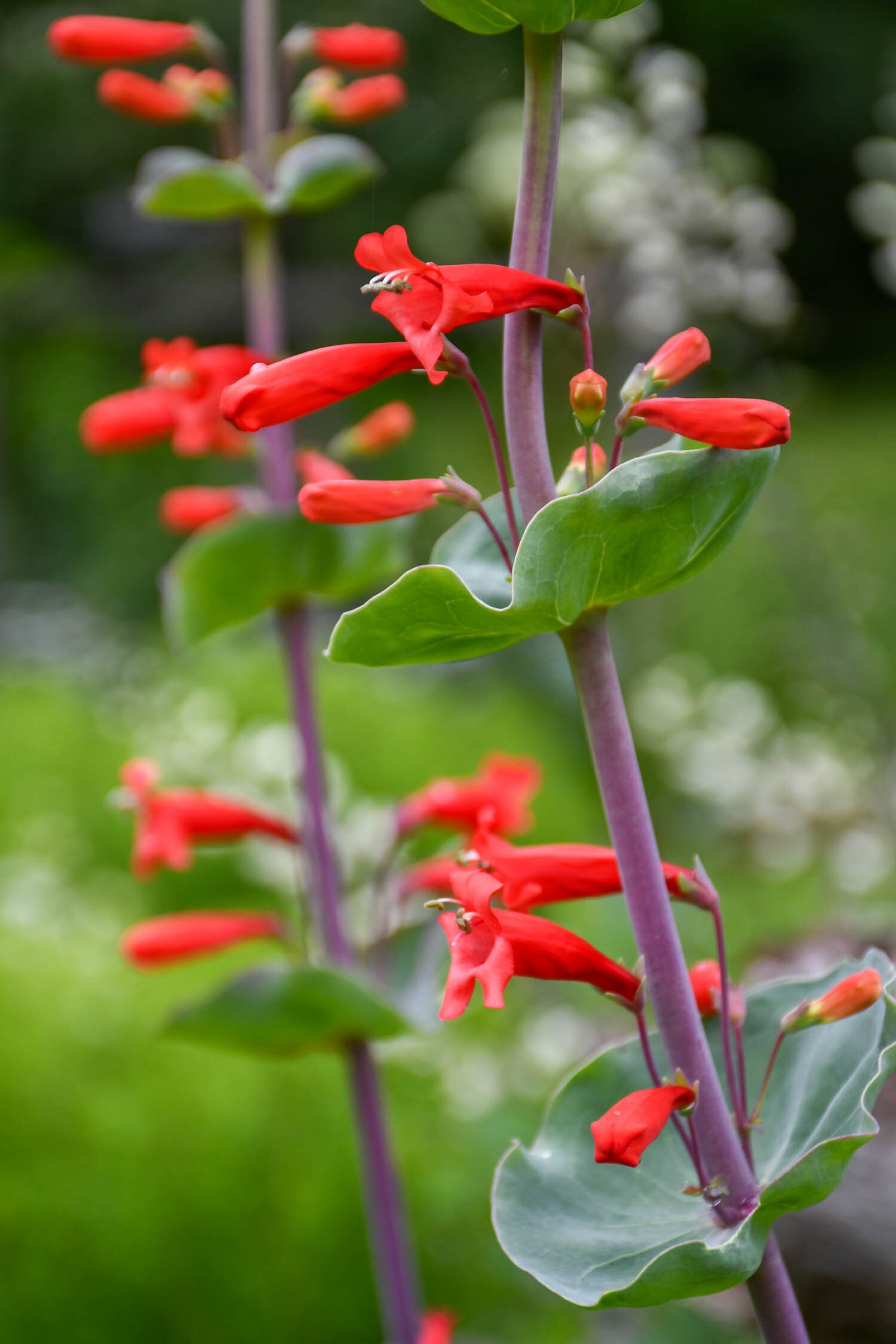This is a full-color, vertically rectangular photograph taken outdoors during the daytime using natural light. The main subject consists of two thick, grayish-purple stems rising upward, with one in clear focus in the immediate vicinity and another, slightly blurred, in the background against a backdrop of out-of-focus vegetation, primarily green with patches of white. The stems are adorned with unique lily pad-like leaves that encircle them, forming bowls that splay slightly upward at the edges. Emerging from these bowl-shaped leaves are striking, red trumpet-shaped flowers. These flowers feature splayed-out petals with grey pods at their centers, adding an unusual and captivating detail to the scene. The overall impression is of a fantastical, almost surreal plant that seems more like a computer-generated image than a natural occurrence.